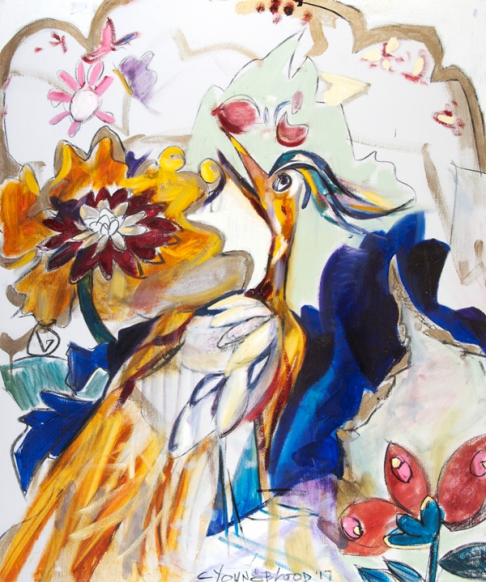A captivating watercolor-like painting signed by C-Y-O-U-N-C-P-H-O-O-D depicts a vibrant bird, presumably a peacock, at the center of the image. The bird's striking head features an array of intricate, spiraling feathers in shades of dark blue, light blue, yellow, and gray, giving it a roadrunner-like appearance. The bird's sharp beak is open, as if poised to consume a nearby berry. The richly detailed tail feathers are a mixture of dark yellow, light yellow, and red.

Surrounding the bird is an abundance of colorful flowers and foliage, creating a lush and almost chaotic abstract background. Prominently to the left of the bird's face, a large, ornate flower with big yellow petals and a red and white center stands out. Smaller pink and purple flowers are scattered around, adding to the vibrant scene. There is also a peculiar, ghost-like shape with red eyes, nestled above the bird, adding an eerie contrast to the otherwise vivid composition. 

In the lower right corner, clusters of leaves or possibly flowers that have yet to bloom present as three large red leaves on flower stems. The entire scene is infused with bright blues, reds, and golds, showcasing the surreal beauty of the peacock intertwined with the luxuriant floral environment.